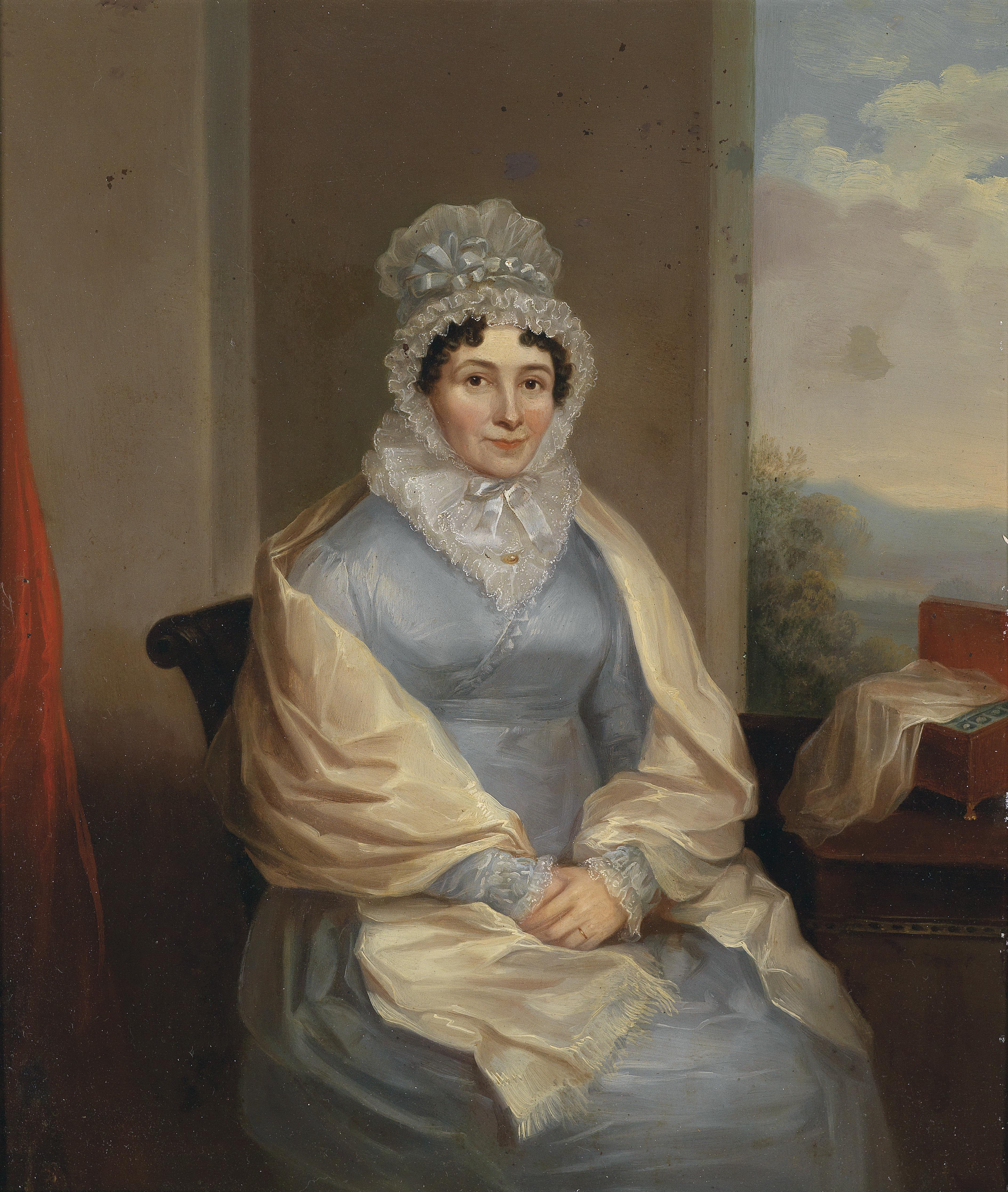This painting, reminiscent of the early 1700s, depicts a woman of possible royalty sitting in a chair beside a table. She is centrally positioned and gazes directly outward with a soft smile. The woman, a white figure with dark brown, curly hair peeking out from an ornate, ruffled white bonnet, wears a long, light blue gown. Draped elegantly over her shoulders is an ivory-colored shawl, while her neck is adorned with an intricate, silver lacy headgear that fully covers her neck. A ring is visible on her left hand, suggesting marital status. 

In the background, a window positioned to the woman's left reveals a cloudy sky with hints of mountains and greenery. The right side of the image features a portion of a red curtain. On the table beside her is a piece of satin fabric atop a container, adding to the painting's detailed texture and rich color palette, primarily consisting of white, blue, tan, and red. The deft use of light and color, coupled with the luxurious fabrics and serene expression of the woman, speak to the affluence and elegance of the period.